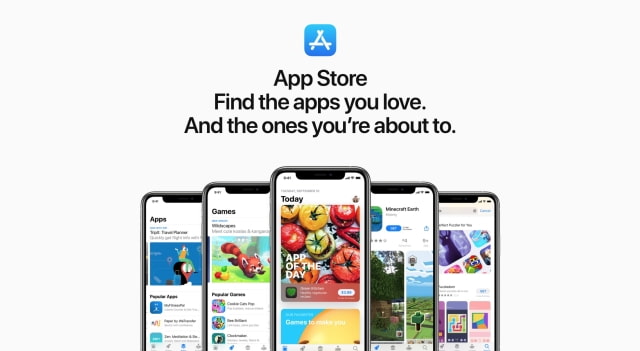This promotional graphic for the App Store features the tagline, "App Store: Find the apps you love and the ones you're about to." The design prominently showcases five iPhone screens displaying various sections of the App Store, including apps, games, and specific recommendations like "Minecraft" and other "Game of the Day" selections. The background is clean and minimalistic, predominantly white, with the standard App Store icon positioned at the very top. Below the tagline, the floating iPhones present a lively and visually appealing representation of the diverse offerings available on the App Store, likely targeting a younger audience with its vibrant and dynamic layout. The devices are strategically placed in a seemingly weightless, gray-white void, reinforcing the sleek and modern aesthetic of the promotional material.